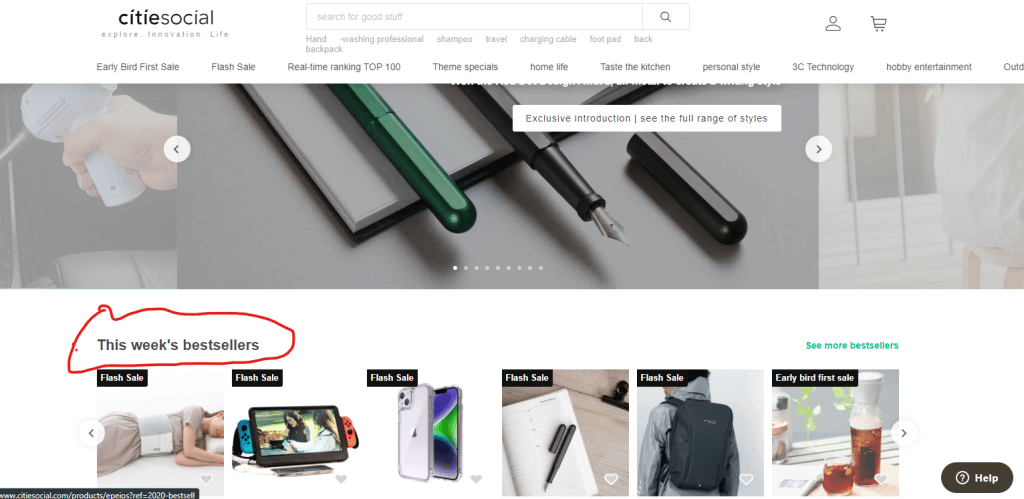Image Caption:
The image depicts a screenshot of a website's user interface. In the upper left corner, there is a title that reads "City Social Explore Innovation Life." Below the title, a search bar displays placeholder gray text that says "Search for good stuff." The site's navigation menu features multiple tabs, including "Early Bird First Sale," "Flash Sale," "Real-Time Ranking," "Top 100 Theme Specials," "Home Life," "Taste the Kitchen," "Personal Style," "3C Technology," "Hobby Entertainment," and a partially cropped tab likely labeled "Outdoors."

Beneath the navigation menu, a rectangular section contains individual slides. One slide features a text box stating, "Exclusive Introduction See the Full Range of Styles." Below this section, on the left side, there is a label with black text declaring, "This Week's Best Sellers," which has been circled in red. Six product images are displayed below, each marked with either "Flash Sale" or "Early Bird First Sale" in the upper left corner. To the far right, a teal-colored button invites users to "See More Best Sellers."